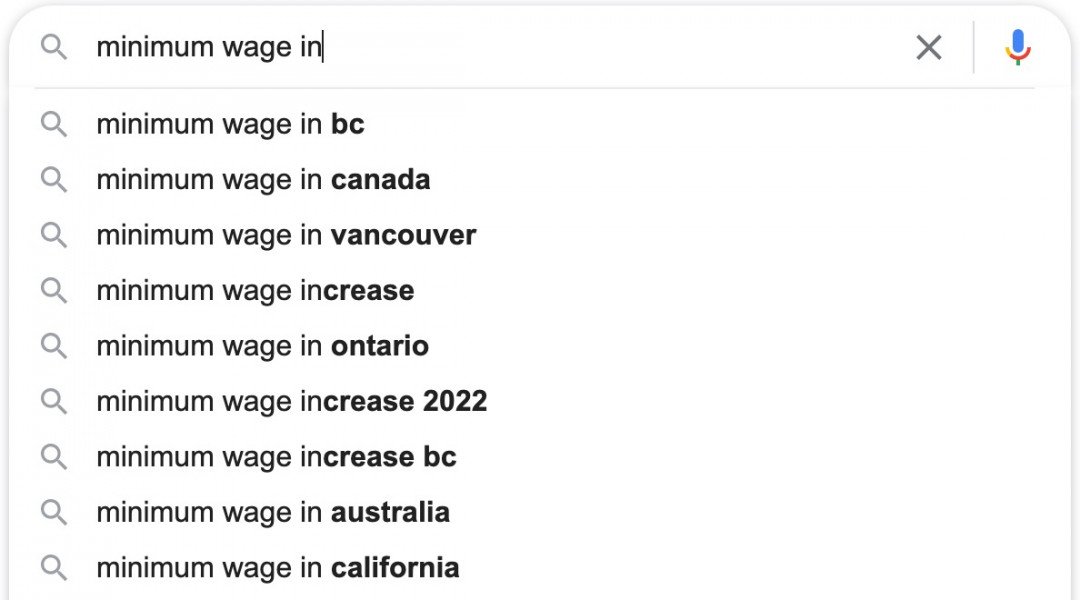The image depicts a Google search page where an individual is in the process of typing a query. Dominating the interface, the iconic Google colors—blue, red, yellow, and green—are visible, along with familiar design elements such as the curved search window at the top and a blue-highlighted microphone icon on the right, indicating voice search capability. Positioned at the uppermost part of the screen, a magnifying glass symbol, representing the search function, underscores the focus on the typed input.

Currently, the query "minimum wage in" is being entered in the search bar. Adjacent to this text entry, there's an 'X' icon for easily clearing the input to start a new search. Directly beneath the search bar, Google offers predictive text suggestions based on the incomplete query. These suggestions appear in a vertical list, each accompanied by a smaller magnifying glass icon. The first suggestion, bolded for emphasis, reads "minimum wage in BC," followed by "minimum wage in Canada" and "minimum wage in Vancouver". The pattern continues with other relevant and popular searches, including "minimum wage increase," "minimum wage in Ontario," "minimum wage increase 2022," "minimum wage increase BC," "minimum wage in Australia," and finally, "minimum wage in California."